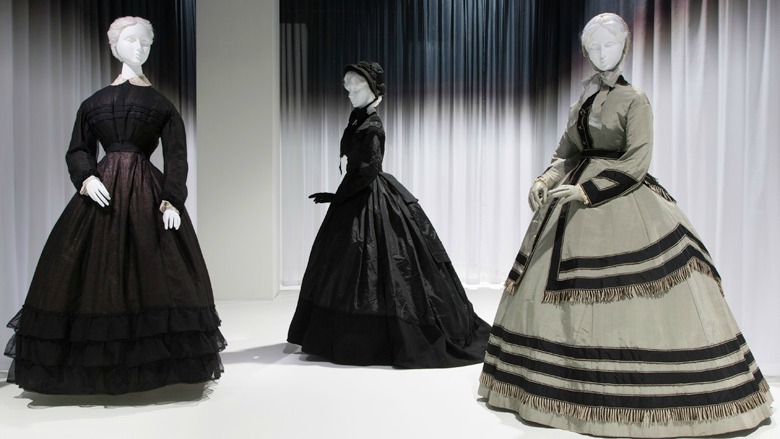In this striking photograph, three meticulously detailed mannequins, each emulating an authentic Victorian style, stand prominently against a backdrop of white curtains that transition to a dark, shadowy black with a hint of blue at the top. The mannequins, white in color with life-like facial features and hands posed realistically, are all dressed in ornate, voluminous gowns.

On the left, the first mannequin is clad in a dark black top paired with a dark pink skirt adorned with three layers of ruffles at the hem. The middle mannequin, appearing to stride forward, wears an elaborate black satin dress with long sleeves and sports a black hat secured under her chin. The mannequin on the right dons a tan dress with comprehensive black lines encircling the bottom, tan fringe beneath the black lines, and black accents on a matching tan jacket. Her headdress, also tan, is tied under her chin, completing the ensemble.

The floor beneath them is a pristine white, complementing the grayscale theme and highlighting the intricate details of their historically inspired attire.